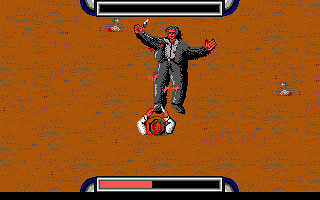A meticulously designed retro-themed video game image features prominently on the screen, evoking a sense of nostalgia. Framed at both the top and bottom edges are classic health bars; the top bar is entirely depleted, rendered in solid black, while the bottom bar is noticeably less than half-full and shaded a vivid red, indicative of the character's precarious health status. The scene is set in a brown, earthy terrain where a central figure strides forward. This character, adorned in a dark gray suit paired with a matching gray shirt, brandishes a knife in his right hand, amplifying the tension.

Dominating the middle of the image, the suited man appears alert and ready for confrontation. Just below him, emerging eerily from the soil, are disembodied arms and a hat, with one arm menacingly clutching a knife, creating a surreal and ominous juxtaposition. The ambiguous nature of the entity—possibly human yet unsettlingly rising from the ground—communicates a palpable threat to the protagonist, intensifying the dramatic tension of the scene.